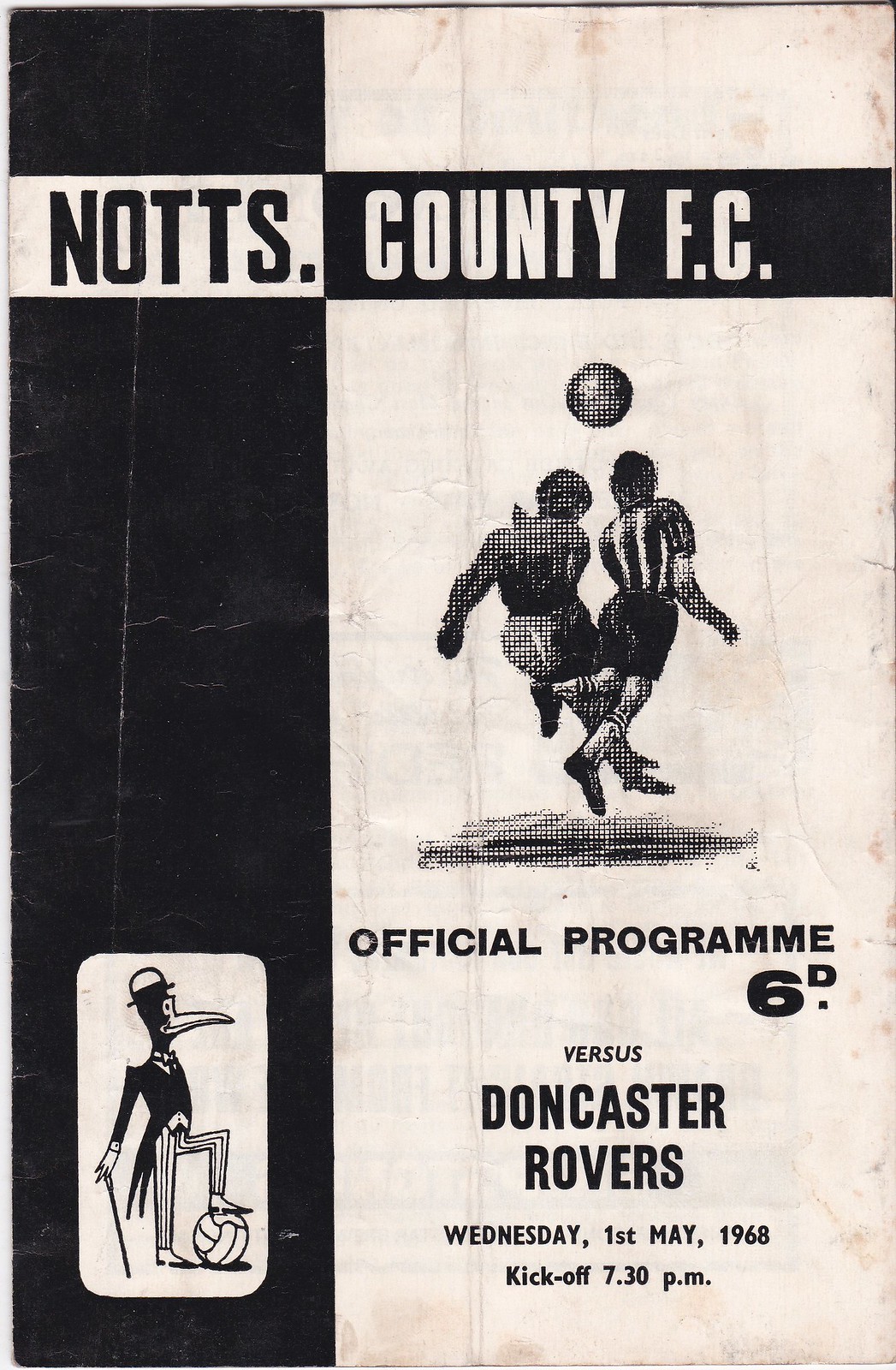This is the cover of an official, aged sports program for a soccer match held on Wednesday, 1st of May, 1968, with a kickoff at 7:30 PM. The program is predominantly black and white, showing signs of wear including folds and water stains. The left side of the cover is black while the right side is either white or off-white, perhaps due to aging. At the top, it clearly states "Knotts County F.C." followed by "Official Programme," spelled with a British "mme" ending. Below the title, it announces the matchup: "Versus Doncaster Rovers." The cover also features a graphical symbol at the top of two players competing for a soccer ball. On the lower left side, there is a charming mascot – a bird that has been described variously as a duck, a crow, or a penguin. This bird, dressed in a fancy tuxedo and hat, is depicted with one foot propped up on a soccer ball and holding a cane in its wing. The price is indicated as "6d," suggesting old British currency. The text is primarily in black except for the word "County" which is highlighted in white.